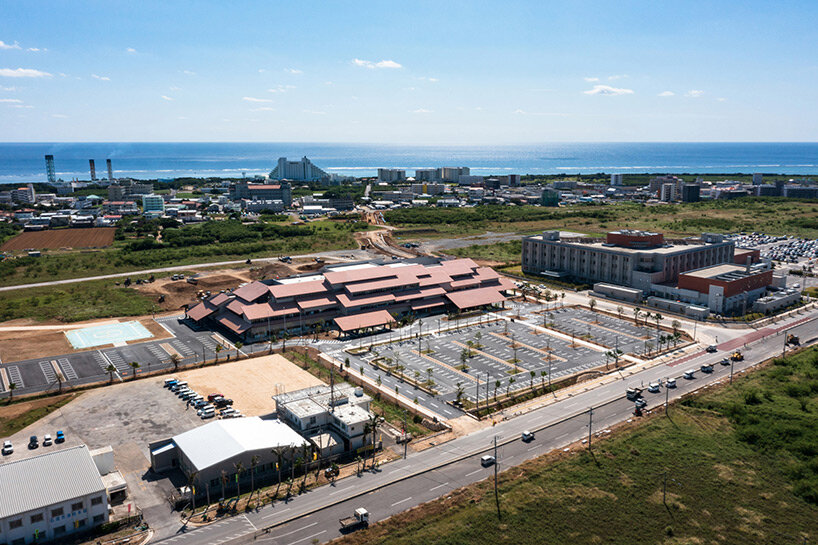In this wide-angle shot of a bustling seaside town or resort, the deep blue sea and the clear, azure sky serve as a picturesque backdrop. Numerous hotels, including a particularly large one that resembles those found in the Bahamas, are visible at the image's far end near the shore. Among the diverse structures, factory towers with steam billowing out can be observed. Centrally located in the frame is an expansive building with multiple roofs, likely a shopping mall, as evidenced by the adjacent, though currently empty, large parking lot. The overall scene captures the serene yet industrious spirit of this coastal locale.